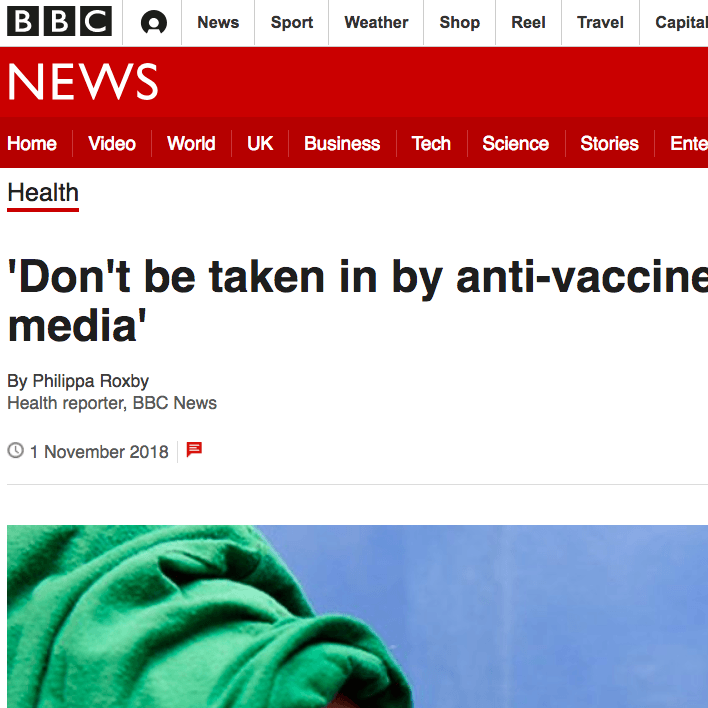This is a detailed screenshot of the BBC news website. The website can be identified as a news platform due to the prominent “NEWS” label displayed in large white text on a red navigation bar. The iconic BBC logo is located at the top-left corner, consisting of three contiguous white squares, each containing one letter of "BBC" on a black background.

Above the main red navigation bar, there is an additional smaller navigation bar featuring an avatar symbol, which likely indicates access to a user profile. This bar contains several categories: "News," "Sport," "Weather," "Shop," "Rest," "Real," "Travel," and another category that is partially cut off and unreadable.

Directly below these navigation elements, the primary red bar reads "NEWS" prominently and it is followed by another navigation bar with categories such as "Home," "Video," "World," "UK," "Business," "Tech," "Science," and "Stories." The final category, "Entertainment," is cut off and not fully visible.

The main highlighted article in the screenshot appears to be health-related, indicated by the “Health” label at the top left with a red underline. The headline reads, “Don't be taken in by anti-vaccine media,” authored by Philippa Roxby.